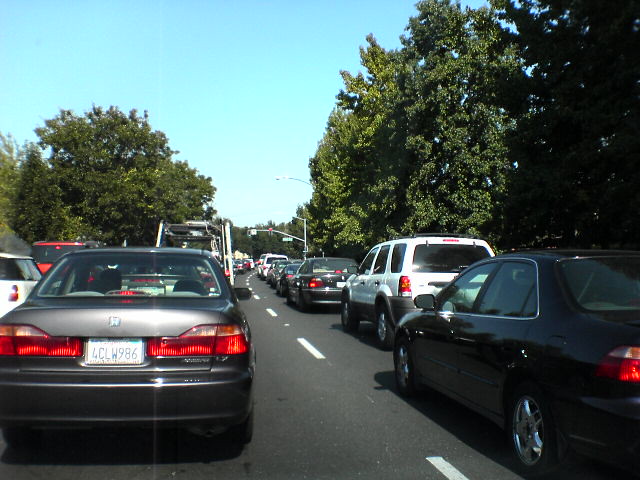This photograph captures a traffic jam on what appears to be a three-lane suburban road, taken from inside a car. The image prominently features two main rows of vehicles, with a visible white-dotted line running down the center. Directly ahead is a gray Honda bearing a white license plate with blue lettering, possibly from California, marked "4CLW986." To the right of the Honda is a black sedan, followed by a white SUV and another dark-colored sedan. A vehicle with a trailer can also be seen in this lineup. On the left, partially visible cars include a red vehicle followed by a white one. The road culminates at a stoplight, which is the cause of the standstill traffic. It is a sunny day with clear skies, and both sides of the road are lined with dense, green-leafed trees, suggesting a lush, suburban setting. This detailed scene is indicative of the early 2000s to mid-2010s based on the car models visible.